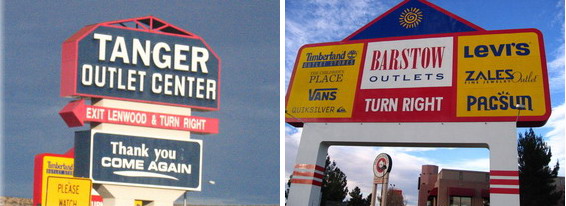The image features two large roadside signs promoting outlet centers, inviting highway travelers to exit and visit. On the right, the prominent sign for Barstow Outlets in California stands out, directing drivers to "Turn Right". It showcases logos for several well-known brands: Levi's, Zales, PacSun, Vans, The Children's Place, and Timberland, with one additional brand that is partially obscured. Beside this sign, the recognizable logo of a Panda Express restaurant is visible, adding to the array of attractions.

The other sign promotes the Tanger Outlet Center, indicating the Exit for Lenwood, and also directing travelers to "Turn Right". The sign kindly ends with "Thank You, Come Again", emphasizing the welcoming atmosphere of the outlet center. Together, these signs create a vivid invitation for travelers to explore the shopping and dining options available at these remote yet bustling retail destinations.